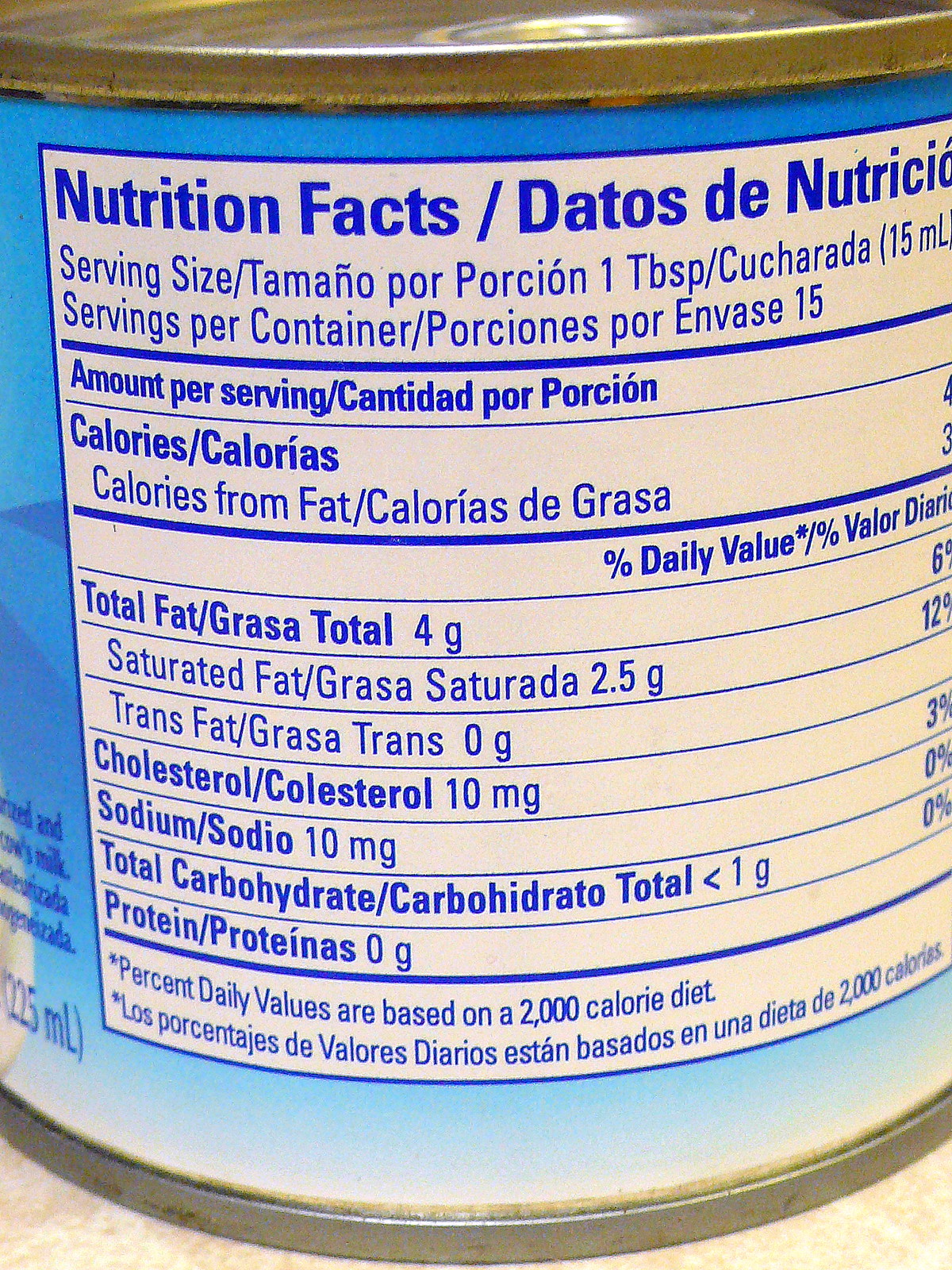This image captures a close-up view of the nutrition facts label on the back of a can of food. The photograph, in color, reveals the can's design dominated by a blue tone. The focus, however, is on the white rectangular box prominently displaying the nutritional information. At the top of the box, bold text reads "Nutrition Facts / Datos de Nutrición," indicating bilingual labeling in both English and Spanish, suggesting the product is either of Mexican origin or intended for a bilingual market. The label provides detailed nutritional data, including serving sizes, calories, total fat, cholesterol, sodium, total carbohydrates, and proteins, among other values.